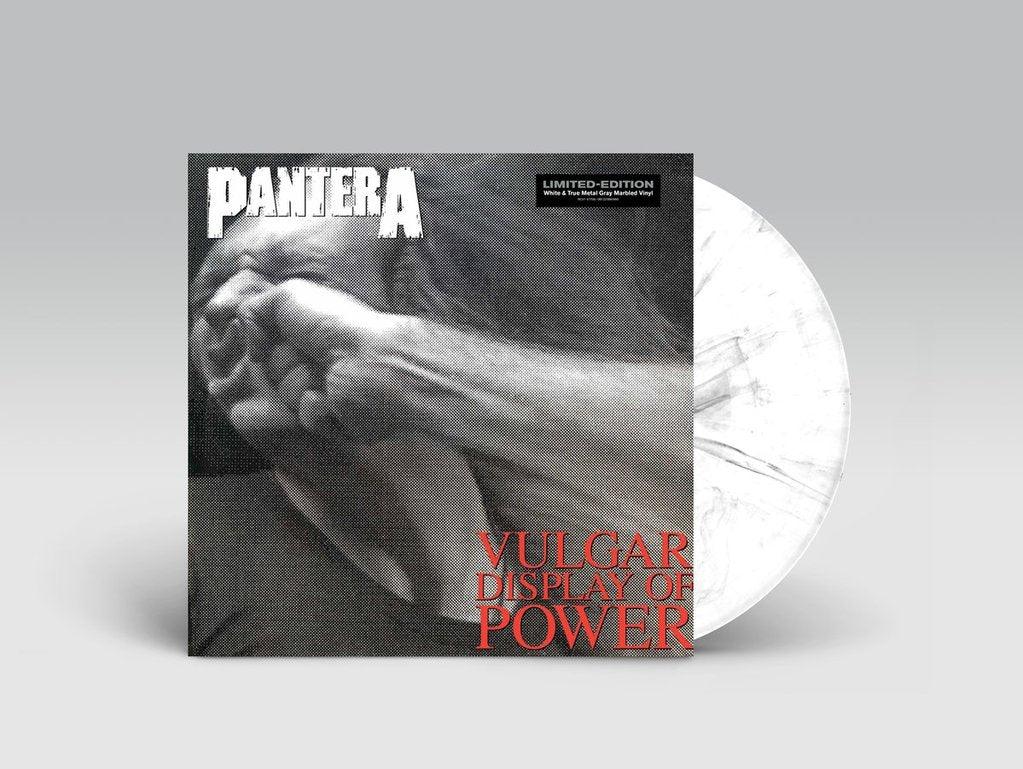This image features the vinyl record of Pantera's studio album "Vulgar Display of Power" set against a gray-white backdrop. In the center of the image is a meticulously scanned representation of the album cover. Dominating the cover is a striking black and white photograph of a man being punched in the face, capturing the moment of impact with intricate details—his cheekbone pushed up, lip curled, and nose scrunched. The assailant's forearm and fist are prominently visible, delivering the right hook.

Across the top of the album cover, "PANTERA" is emblazoned in bold white letters, with the 'P' larger than the subsequent characters. To the top right, within a black horizontal rectangular box, the text "Limited Edition" is noticeable along with additional information about the songs. At the bottom right, the album's title, "Vulgar Display of Power," stands out in striking red text. The cover also features a distinct grid-like texture overlay.

Protruding from the side of the vinyl image is a glimpse of the record itself, styled with a white and grayish marbled appearance. All these elements are positioned against a plain gray backdrop, enhancing the dramatic visual of the album art. The person in the photograph appears to be wearing a grey t-shirt, and their hair flows with the motion of the impact.